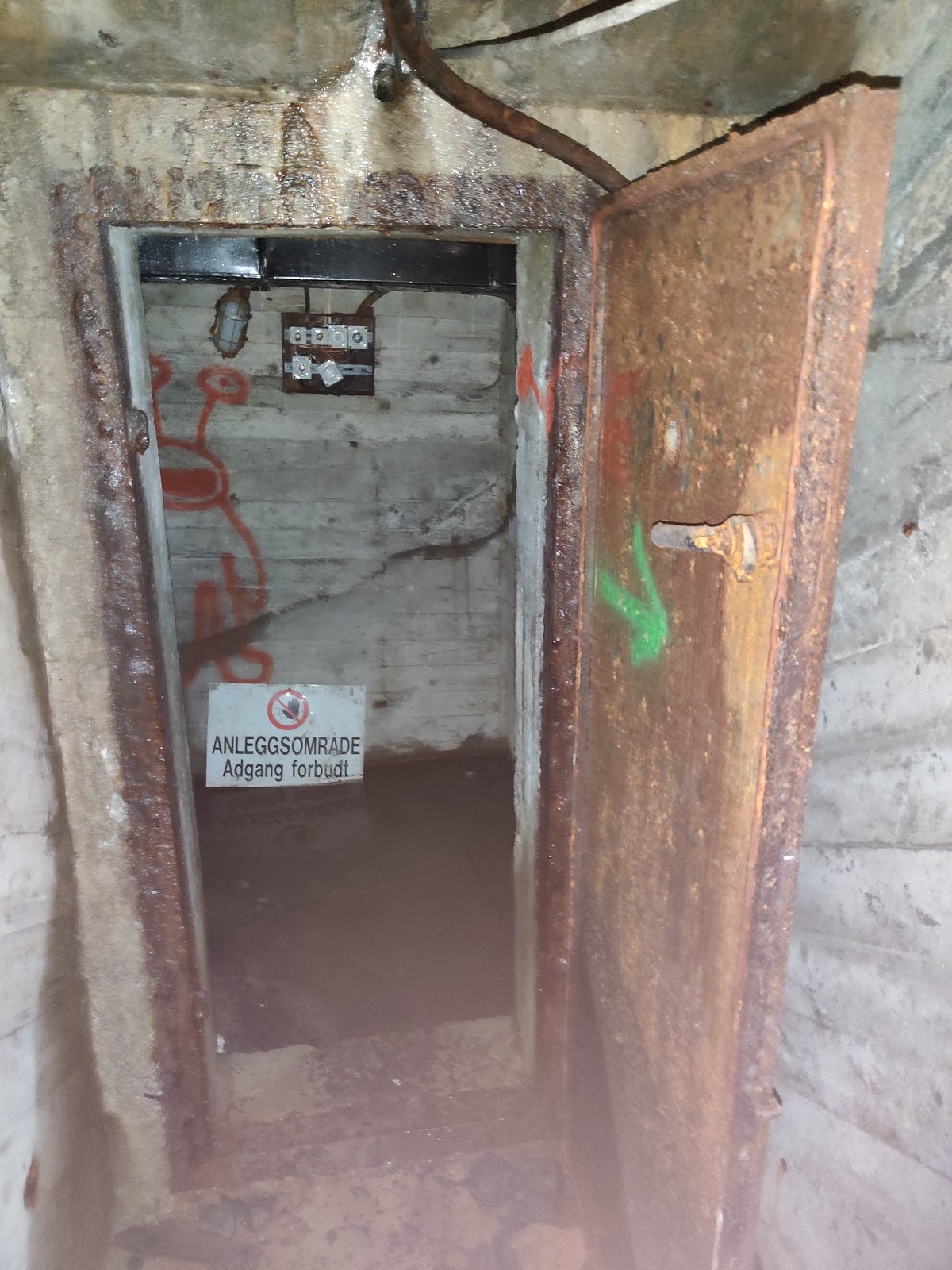The image portrays a narrow hallway constructed from white and gray stone, resembling a bunker or cave. At the end of this corridor stands an old, rusted metal door that is slightly ajar. The inside of the door features a green spray-painted arrow and a rudimentary handle. Beyond the door, the space appears to be reinforced with additional stone walls. The interior of this area functions like a small, cluttered room or closet. On one wall, a black control panel with silver knobs is visible, partially obscured by red spray paint, which forms an alien-like character. The floor of this room is covered in dirt and mud, adding to the sense of neglect and decay. A white sign with black text in a foreign language, potentially German, lies discarded on the ground. It also features a symbol of a hand inside a red circle with a line through it, indicating a prohibition. The overall atmosphere is that of an old, abandoned bunker-like structure with elements suggesting secrecy and restricted access.